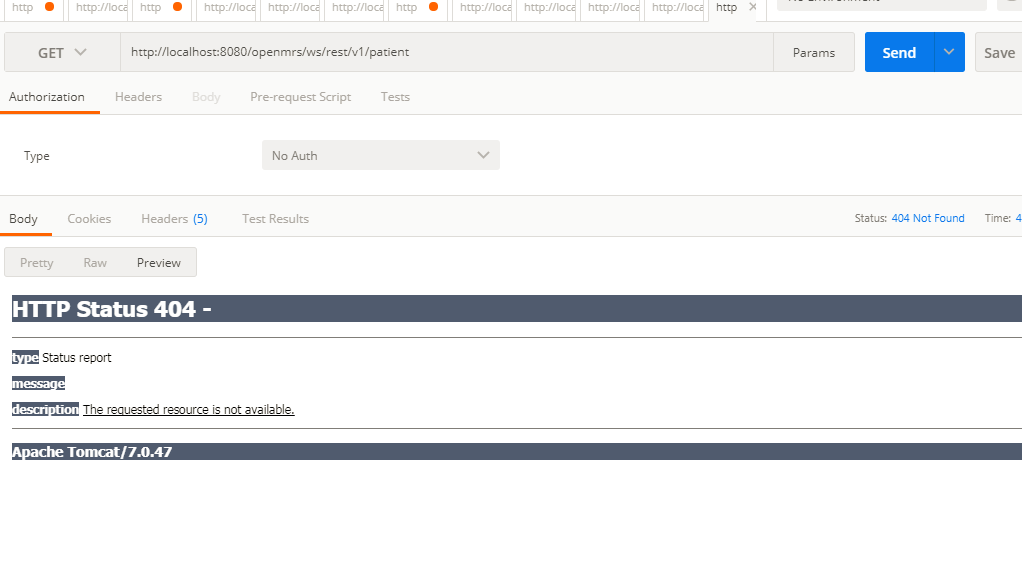In the image, we see a web browser displaying a console or web page interface with 12 open tabs. The address bar contains the URL "http://localhost:8080/openmrs/ws/rest/v1/patient." The interface includes various sections labeled "Authorization," "Headers," "Body," "Pre-request Scripts," and "Tests." The color scheme consists of a predominately white background, accented with blue, orange, and black elements. The layout suggests it could be a developer environment or a testing tool, likely for interacting with the OpenMRS API.